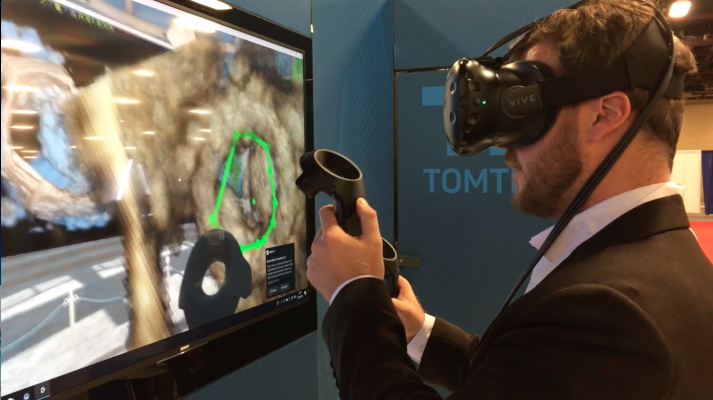This color photograph, taken indoors at what appears to be a convention or trade show, depicts a man engrossed in a virtual reality experience. The man, dressed in a black suit with a white collared shirt, is equipped with a VR headset identified by the "Vive" logo. The headset features a wide black band narrowing as it approaches his face and is secured with a strap around his head. In his hands, he holds two black motion-sensing controllers, each featuring a circular design with handles. 

To his left, there is a large wall-mounted TV screen displaying a somewhat blurry map or diagram highlighted by a green circular area. The backdrop of the scene includes a partially visible door marked with the beginning letters "Tom T," hinting at the setting being a spacious convention hall. The man appears to be manipulating images on the screen, possibly related to bones or skeletal structures, indicating that he is deeply engaged in a virtual reality simulation or interactive exhibit in this bustling trade show environment.